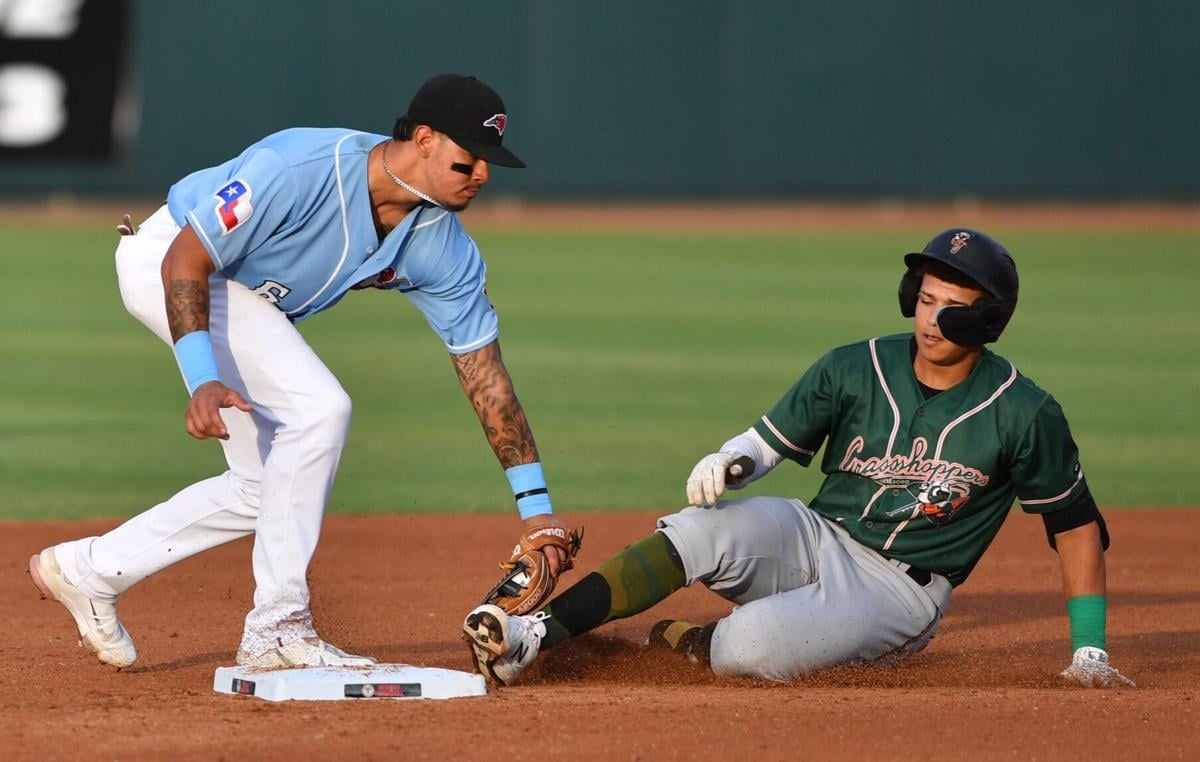This photograph captures a close play at a baseball game, most likely from a minor league or an unaffiliated league. The focal point is a player from the team "Grasshoppers," dressed in a green jersey, gray pants, black helmet, and green and black socks, sliding into a base. His left arm supports his body as his right foot nears the base while the baseman, clad in a sky blue jersey with a Texas flag, white dirt-stained pants, white shoes, and a black cap, reaches down with his glove to tag him. The scene is tense with the baseman's glove just inches away from the sliding player's foot, which appears to be right on the edge of the base, leaving the outcome of the play uncertain. The dirt kicks up around them, highlighting the athleticism and hustle of both players.